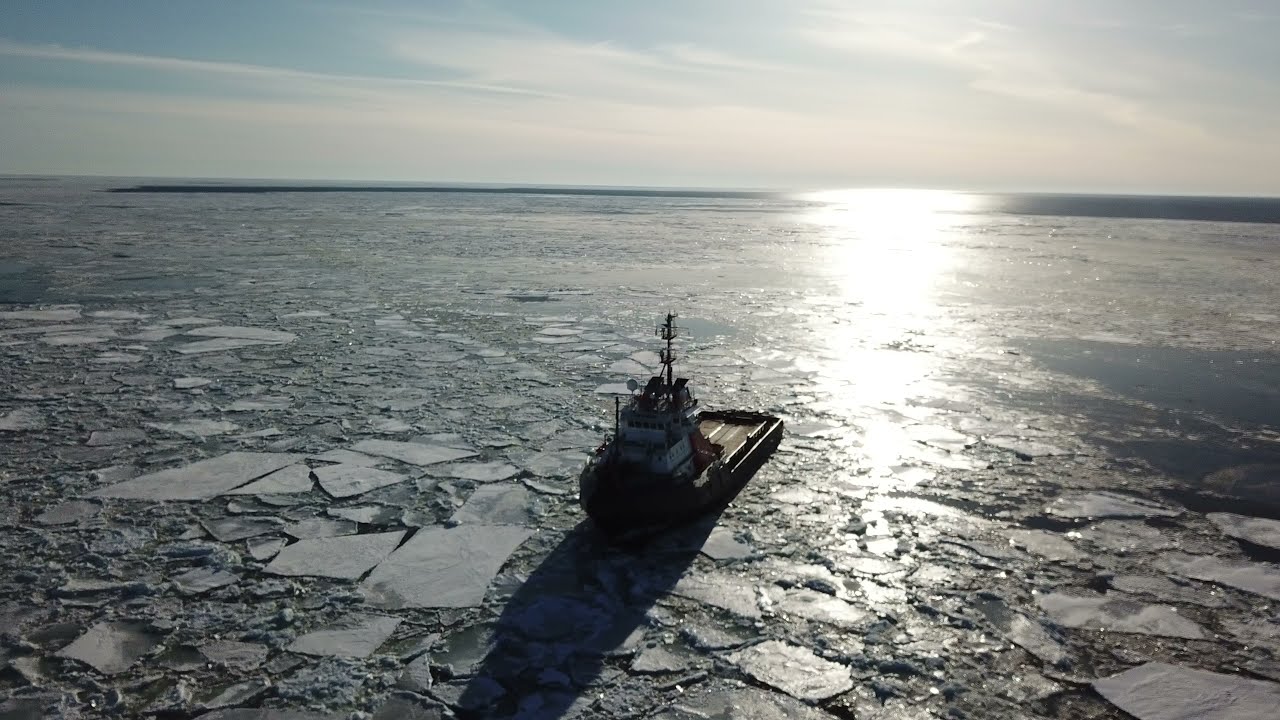This photograph, taken at what appears to be early in the day, captures a large body of water, likely the ocean or sea, under a blue sky with light, blending clouds. A sizable boat, resembling either a Coast Guard cutter or a large fishing vessel, is central in the image. This boat—featuring a white cabin and possibly rubber around its frame—sails through a frigid expanse of water filled with substantial, often square or rectangular chunks of ice. The ice, looking as if it was shattered from a once solid sheet, spreads across the water surface, with no visible people on the ship. The sunlight's diffuse glow reflects subtly on the icy water, enhancing the cold and pristine atmosphere of the scene.